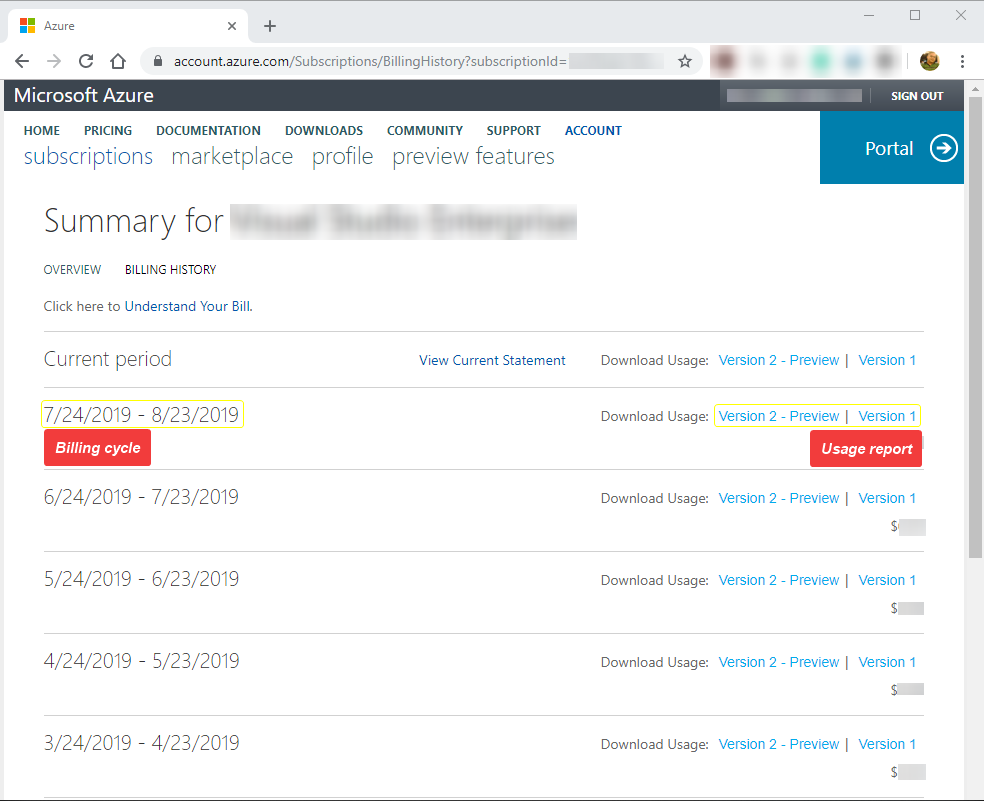The image depicts an open window in the Microsoft Edge browser, showcasing a detailed view of a specific webpage. At the top of the window, there is a light gray header leading into the browser tab on the left. The tab features the Microsoft logo, comprised of four distinct squares forming a larger square: a red square in the top left, a green square in the top right, a blue square in the bottom left, and a yellow square in the bottom right.

Directly below the tab bar, there is a dark gray back button. To its immediate right, a light gray forward button that is disabled, indicating that there are no forward page navigation options available. Next to the forward button is a dark gray refresh icon, and adjacent to it is a similarly colored home icon.

Continuing right, there is an elongated URL address bar with a light gray background. The URL displayed is account.azure.com/subscription/billinghistory?subscriptionId=, with the subscription ID part blurred out for privacy. All icons to the right of the URL bar are also blurred out.

Below the address bar, a header features a gradient starting from black on the left and fading to gray on the right. It displays "Microsoft Azure" in white lettering. 

Underneath this header, a navigation menu on a white background presents several options in dark gray or black font: Home, Pricing, Documentation, Downloads, Community, Support, and Account, with the 'Account' option distinguished in blue.

Further down, another lighter, more circular font lists additional options: 'Subscriptions' in blue, followed by 'Marketplace,' 'Profile,' 'Preview,' and 'Features' in gray. Lastly, a prominent dark gray or black text reads "Summary for" followed by a blurred-out area.